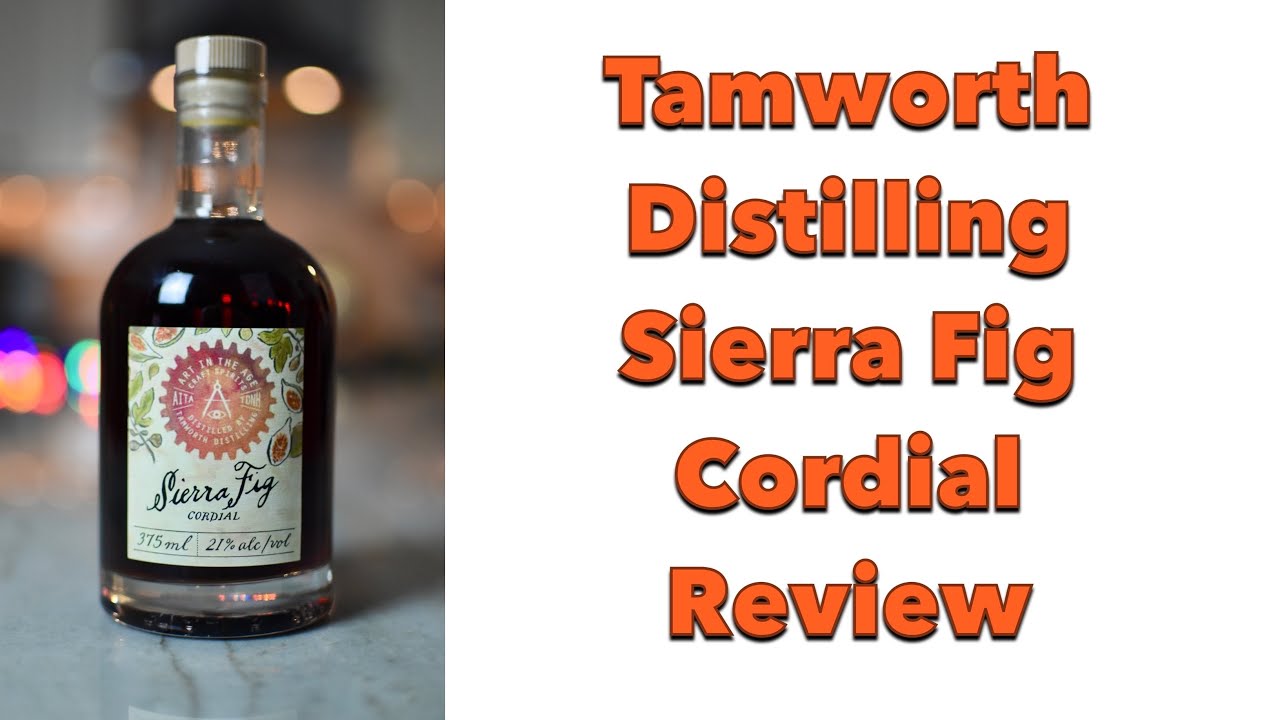In the image, we see a vertical rectangular picture prominently featuring a bottle of alcohol on the left side and centered text on the right side, both against a solid white background with no border. The bottle, which holds a deep red liquid, has a clear glass body and a light brown grooved screw cap. The front label of the bottle is primarily beige and displays the product name "Sierra Fig Cordial," along with the volume "375 ml" and alcohol content "21% alk/vol." The label also features green leaves and white and brown illustrations, likely representing figs, all set around a pink and gray gear-like design. The label includes the text "Art in the Age Craft Spirits, Distilled by Tamworth Distilling." The bottle rests on a white countertop with light gray marble or granite lines and spots. The background behind the bottle is blurry, showcasing a mix of yellow, white, dark blue, light blue, red, pink, green, and orange lights, adding a warm, ambient feel. The right side of the image displays block-style orange letters that read: "Tamworth Distilling, Sierra Fig Cordial Review."